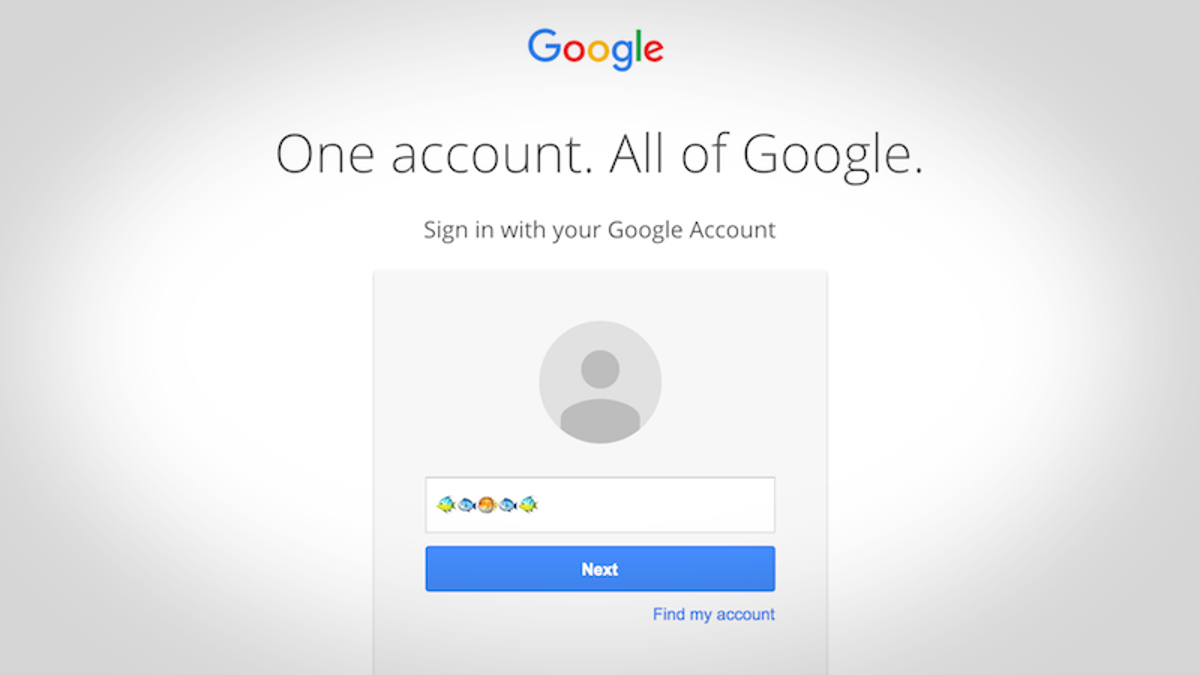Displayed is the Google sign-in screen, which is the initial interface encountered when accessing Google for the first time. The screen has a predominantly gray background, with a white highlighted section in the center. At the top, the iconic Google logo is prominently featured, consisting of the word "Google" in various colors: a blue "G," a red "O," a yellow "O," another blue "G," a green "L," and a red lowercase "e."

Beneath the logo, a large, black, non-bolded text reads, "One account. All of Google." Following this, there is a prompt that says, "Sign in with your Google Account."

In the middle of the screen, there's a secondary gray box that houses a small thumbnail area meant for your avatar or personal photo, if you have one added to your account. Adjacent to this, there is a small text box where users can type their password. Below this input area is a blue rectangular button with the word "Next" written in white font, facilitating the continuation of the sign-in process.